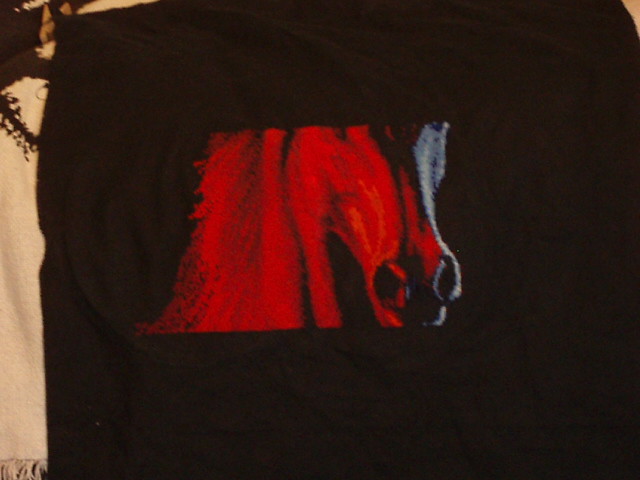This image features a slightly grainy photograph of a black, wrinkled article of clothing, most likely a sweatshirt or t-shirt, which appears to be laying on a white surface. The centerpiece of this clothing item is a red, partially viewable horse head graphic. The horse's face is prominently displayed, with the image cutting off just above the eyes and just below the nostrils, leaving the small visible portion of its lips partially visible. The horse's neck and mane are also visible. The side of the horse facing the camera has a red tint with maroon hues around its mane, while streaks of black and dark gray accentuate its nose and neck. The right side of the horse’s face transitions into dark gray with light gray streaks, giving a split-toned effect. The surrounding white surface peeks through on the left side, showing a strip of the white material with a small black design at the top. The overall presentation hints at possible graphic design origins, where the clarity of whether it’s a photograph or AI-generated remains ambiguous.